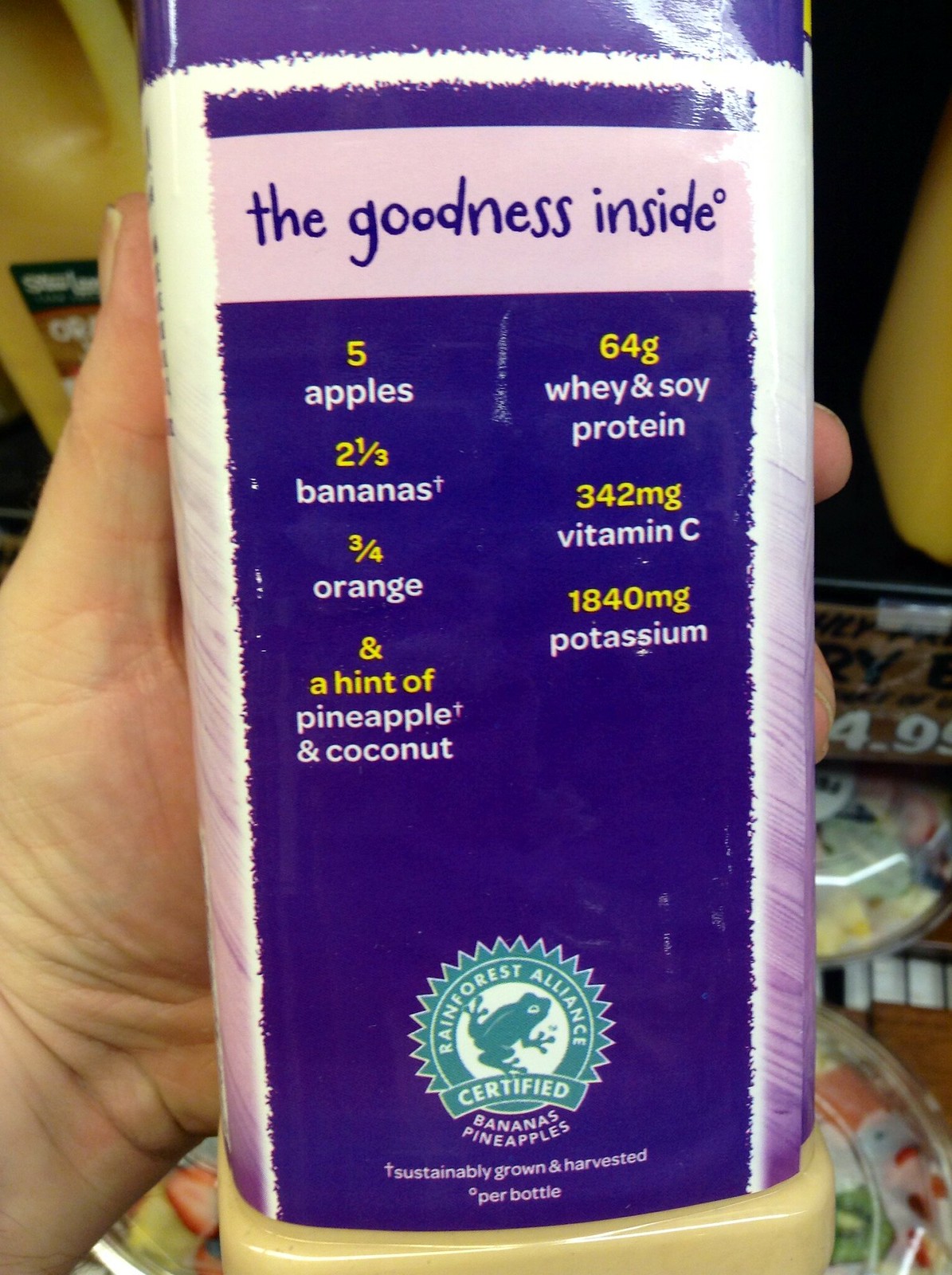The image is a photograph of a hand holding a predominantly purple bottle with a label featuring a mix of white details. The label prominently displays the phrase "The Goodness Inside" in purple text. Below this, there is a detailed list of the drink's ingredients and nutritional content: 
- Five apples
- Two and one-third bananas
- Three-quarters of an orange
- A hint of pineapple and coconut
- 64 grams of whey and soy protein
- 342 milligrams of vitamin C
- 1,840 milligrams of potassium

At the bottom of the label, there is a green and white emblem resembling a metal badge, indicating "Rainforest Alliance Certified" with a frog icon at the center, surrounded by a ribbon-like design. Beneath this badge, the label specifies that the bananas and pineapples used in the beverage are sustainably grown and harvested.